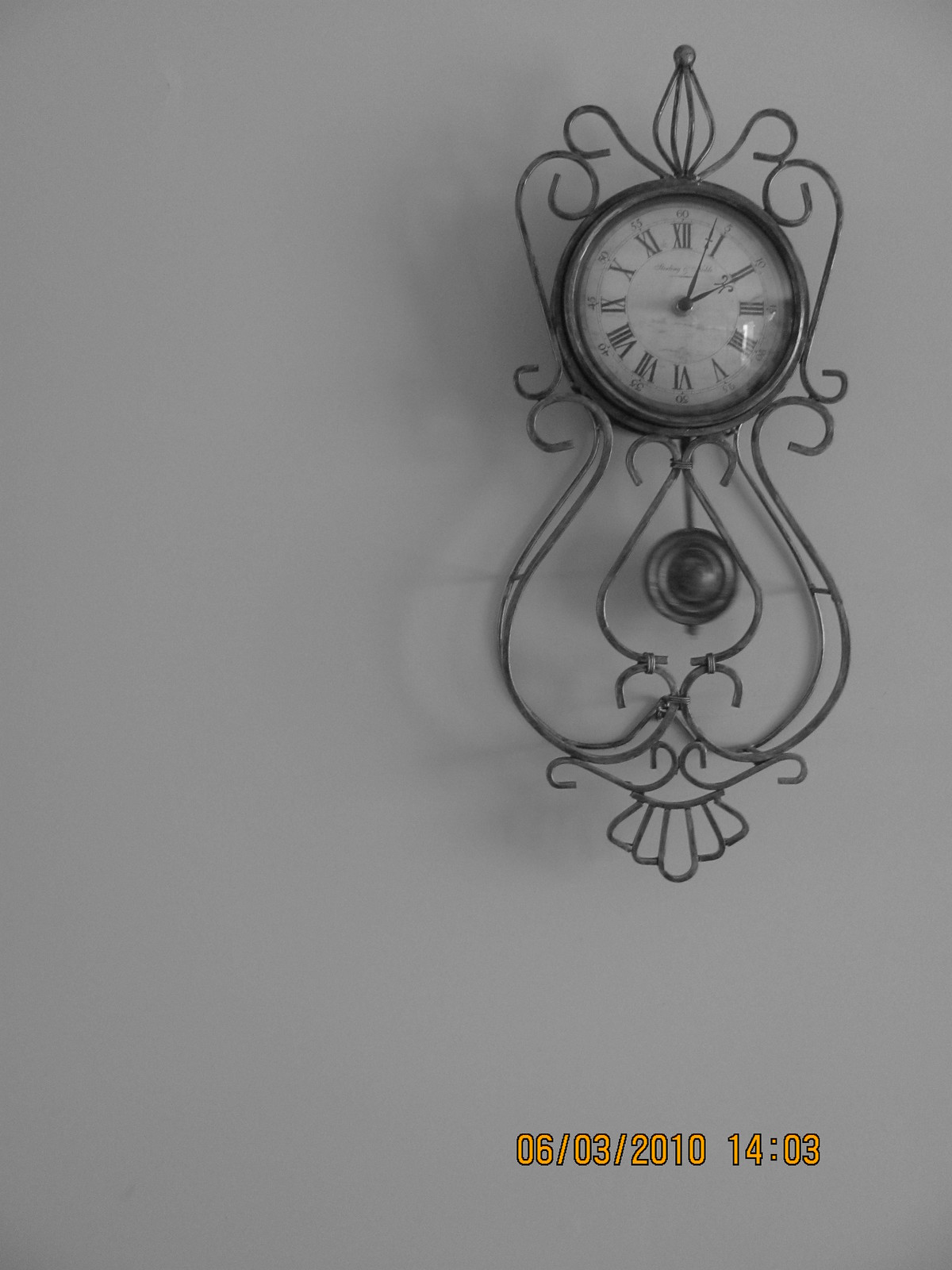A photograph depicts an ornate wall clock mounted against a dark grey backdrop. The clock features an intricate design with elegantly bent metal that curves gracefully around a solid, circular metal frame encasing the timepiece. The face of the clock displays Roman numerals to indicate the hours, while the center showcases delicate clock hands. The clock's face includes a name or signature, although it is partially obscured, making it difficult to read. Below the clock's hands, there is another clearly visible signature. The clock, moderately small in size, is embellished with decorative, curled metal wires that add to its ornate appearance. A date and time stamp at the bottom of the image reads "06-03-2010, 14:03."